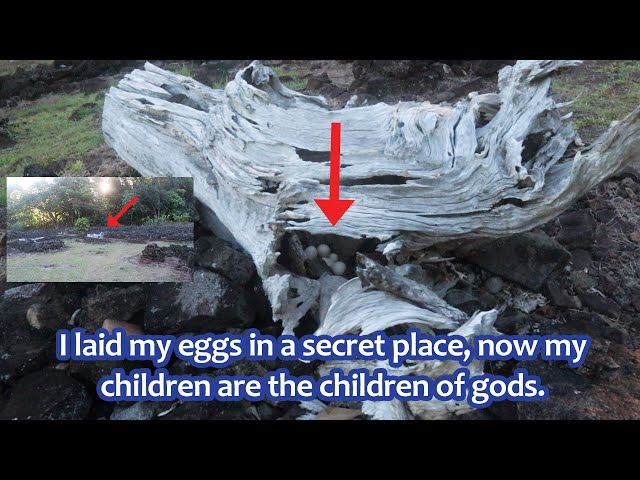The image showcases a close-up of a driftwood stump located on a rocky beach or bank, surrounded by a body of water and backed by trees with sunlight filtering through. In the forefront, there is a cut-out section on the left side that provides a further back angle, revealing the log's location. Notably, the log holds hidden eggs, highlighted by a red arrow pointing downward. White text outlined in blue, and in a serif font, reads: "I laid my eggs in a secret place, now my children are the children of the gods." Although the species of the egg-laying animal is not identified, the composition also includes a small green bush near the log and a white torn cloth partially covering the eggs, adding an element of mystery and intrigue to the scene.